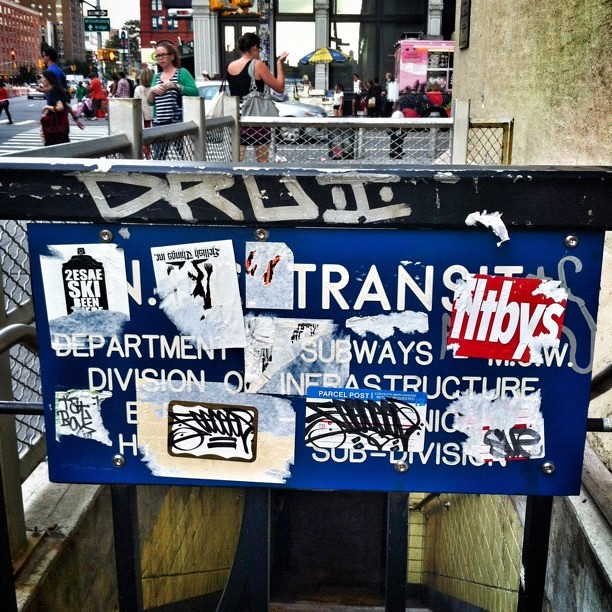The digital photograph depicts a densely crowded urban street scene dominated by a blocked-off subway stairwell encircled by a silver fence and railing. The stairwell area is overlaid with a blue sign featuring white text that reads, "Department Subways Division of Infrastructure," partially obscured by graffiti and stickers, including ones that reveal the word "transit" marred by a sticker reading "NTBYS" and graffiti spelling "D-R-U-I." The bustling backdrop reveals a busy intersection teeming with people navigating the sidewalks and crosswalk, alongside buildings, cars, and a hot dog vendor. The mixed palette boasts royal blue, red, white, black, yellow, tan, gray, green, and pink tones, which contribute to the image’s chaotic and vibrant atmosphere.